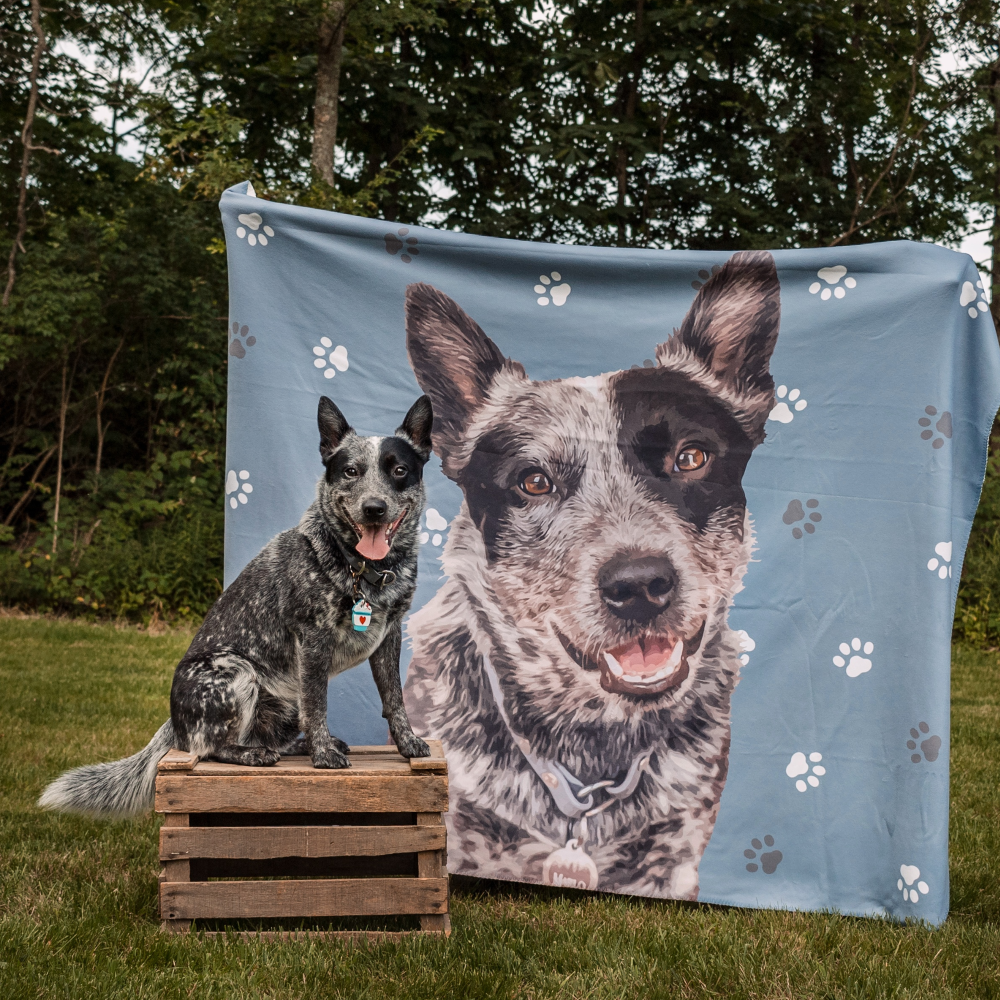In this charming photograph, a large, mixed-breed cattle dog, sporting a coat of gray, black, and white spots, sits proudly atop a wooden crate. The dog, resembling the size of a German Shepherd, has perky black ears and a collar with an unidentified tag dangling from it. The dog’s open mouth and hanging tongue give the appearance of a happy, smiling expression. Positioned directly behind the dog, a person—concealed from view—holds up a large blue blanket adorned with little paw prints and a central image of the same dog’s face. The photograph is set outdoors in a lush, green backyard with tall trees forming the backdrop. The overall ambiance suggests a slightly overcast day, adding a soft, natural light to this adorable scene.